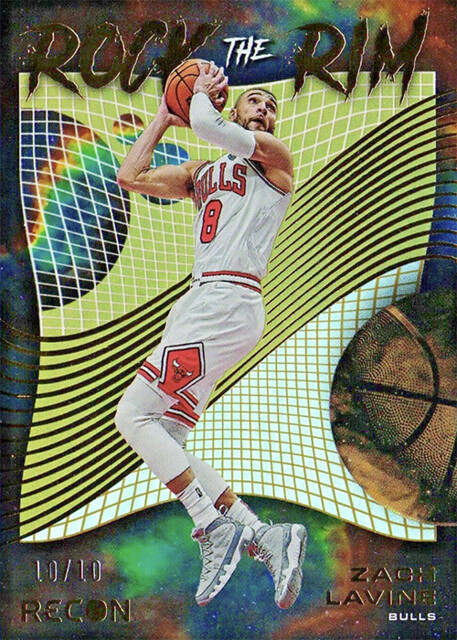This vertically aligned rectangular image depicts a basketball player soaring through the air, preparing for a shot. His body is mainly facing left, although he is slightly turned away from us, cradling a basketball between both hands near his face. The player is clad in a striking white and red uniform emblazoned with the word "Bulls" in red letters across the chest and featuring a red number eight. Above the player, bold text reads "ROCK THE RIM," with "ROCK" and "RIM" in dark brown and "THE" in white, all in uppercase letters.

The background is a vibrant blend of green, orange, red, brown, and blue hues, creating a dynamic visual frame around the player. Directly behind him is a distinct, curved square shape, suggestive of a globe, adorned with rainbow-colored landmasses, and marked by diagonal curved lines descending from left to right. Additionally, the lower right corner of this shape features a checkered pattern of light brown and white squares.

On the right side of the image, only the top half of a basketball is visible, marked with black lines against its brown surface. The lower left-hand corner of the image bears the inscription "10/10 Recon," while the lower right-hand corner identifies the player: "Zach LaVine, Bulls."